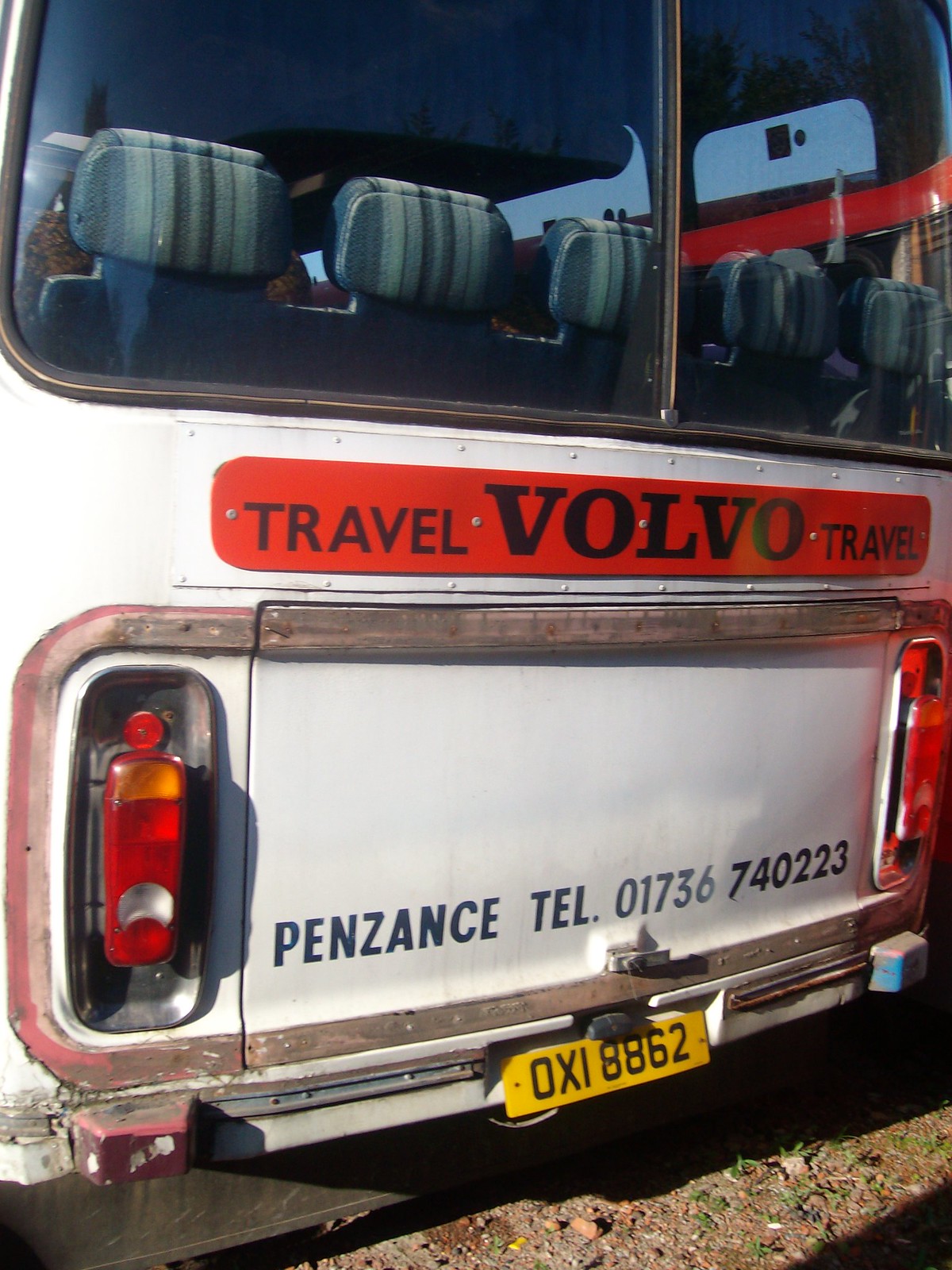This photograph captures the rear view of a parked white bus, situated on a rocky dirt surface outdoors. Prominently displayed is the European license plate, OXI-8862, which is yellow and situated below a printed sign that reads “Penzance TAL 01736 740223”. The bus features clear, non-tinted rear windows through which the rear row of five striped seat backs is visible, yet no passengers are present. Positioned above the taillights is an orange sign with black text stating “Volvo Travel”. The bus's stoplights are also clearly seen, emphasizing its stationary position.